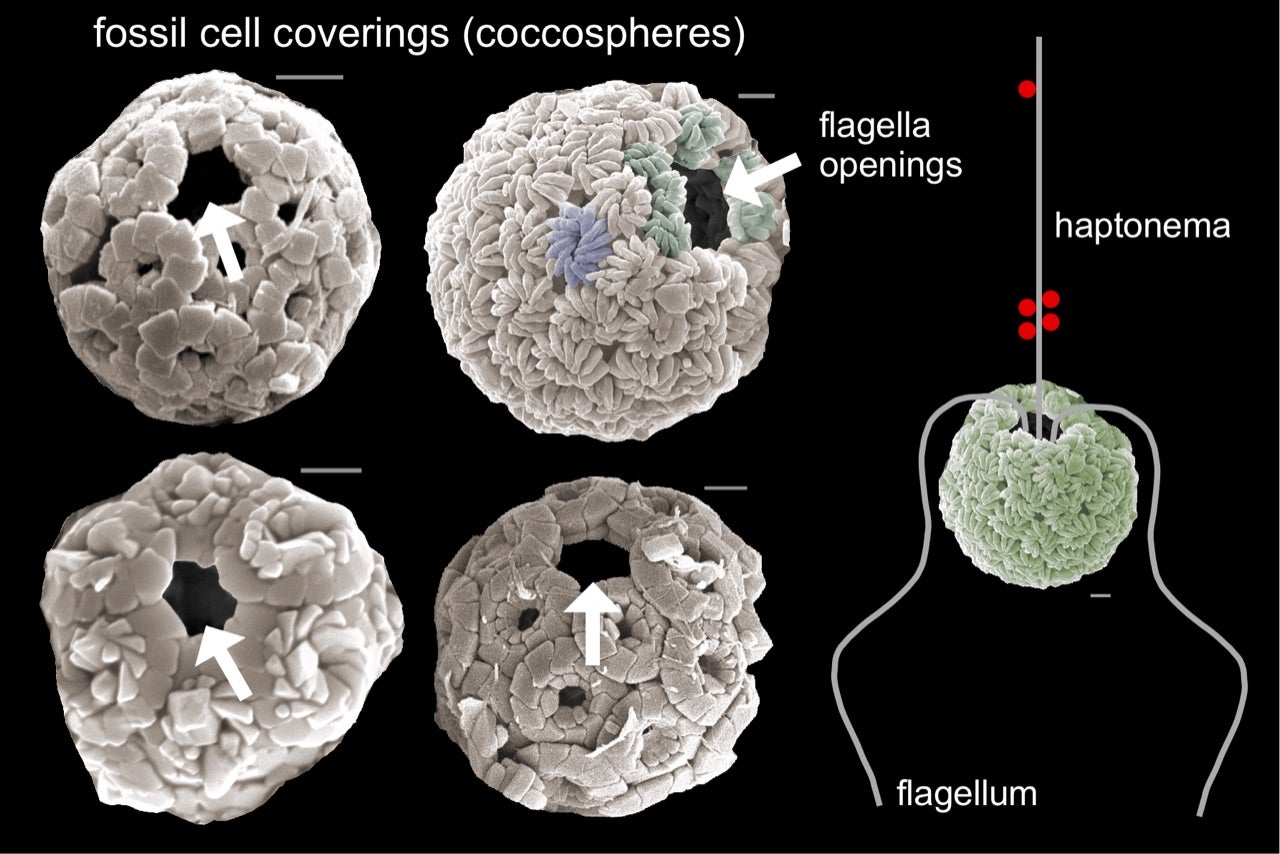On a black background, the diagram displays various schematic representations of fossil cell coverings, labeled in white at the top left as "Fossil Cell Coverings (Cocospheres)." This white text heads a chart that meticulously illustrates four distinct types of fossil cell coverings, each comprising white circular or patterned objects. 

- At the top left, a sphere comprised of structures resembling pineapple slices has a white arrow pointing up and to the left towards a visible gap.
- To its immediate right, a similar sphere, distinguishable by its arrangement akin to pasta shells, features an arrow from the upper right side pointing down and to the left towards another gap, with the label "FLAGELLA openings" next to it.
- Below the first sphere, another arrangement likened to gathered pineapple slices shows a white arrow in the middle pointing upward towards an opening.
- The final depiction on the bottom left resembles clustered rocks, with a white arrow also pointing towards an open gap.

To the right of these illustrations, a vertical white line connects the top of the diagram to the center of a spherical depiction, adorned with one red dot at the top of the line and four red dots at the bottom split to the left and right. The label "HAPTONEMA" is positioned to the right of this vertical line. Additionally, this central sphere has lines extending outward; the left line curves down in a left-then-right pattern, and the right line extends outward before descending in a right-then-left manner. The label "FLAGELLUM" is noted in the lower right corner of the diagram. 

The collective elements of spheres, arrows, and annotated gaps intricately describe the varied structures and functional openings within fossil cell coverings known as cocospheres.